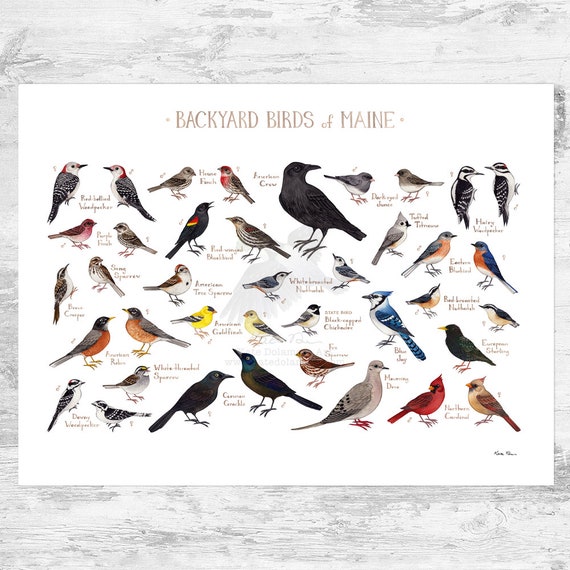This image is a detailed, illustrated poster titled "Backyard Birds of Maine," set on a white piece of paper that overlays a background resembling white-painted wooden boards. The title, written in brown, heads the poster and spells out Maine, M-A-I-N-E. The poster features around 40 different birds indigenous to Maine, each illustrated with names next to them.

To the top left, we see a bird with a distinct red head and black speckled wings identified as a red-headed woodpecker. Directly below are a black and gray finch and another finch with a red chest and black and white markings. The largest bird, placed prominently in the center, is an all-black crow looking to the right. In the top right corner, another woodpecker with a white chest and black wings speckled with white is illustrated.

Among the myriad of birds depicted, notable mentions include a sparrow that is widely recognizable, a vibrant yellow goldfinch, a blue jay with striking blue plumage, and brightly colored cardinals. Additionally, a tree sparrow is positioned to the left. The various birds are portrayed in different directions, enhancing the dynamic nature of the poster, which serves both as an informative chart and a visually engaging tribute to Maine’s backyard birds.